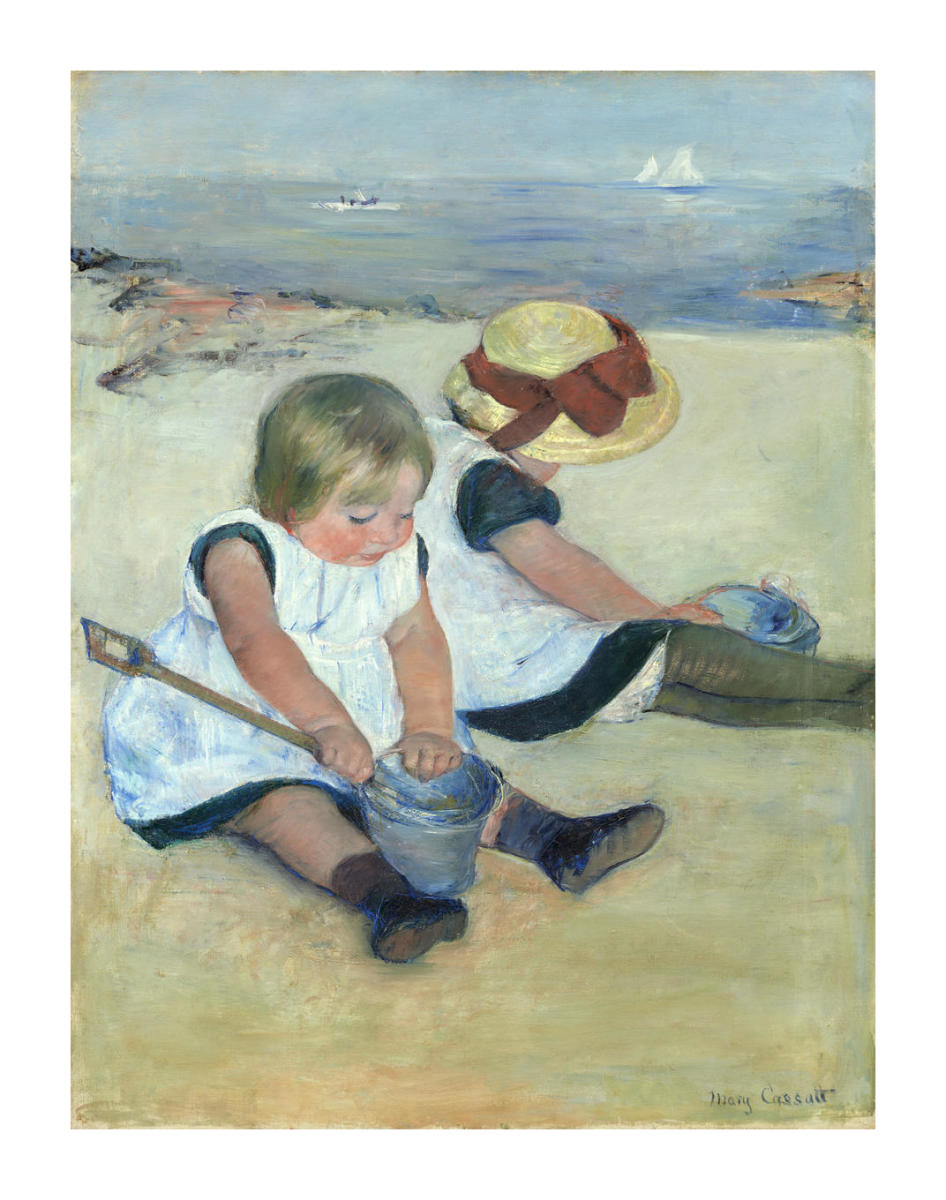This detailed painting by Mary Cassatt, titled "Children at the Beach," depicts two young girls, likely toddlers, seated on the sandy shore, away from the ocean's edge. The painting captures an old-fashioned charm with the girls donning dark dresses and white pinafores. Both girls have black boots, with one wearing dark socks and the other dark tights.

The girl on the left, who has short blonde hair and rosy cheeks, faces the viewer, her round face full of innocence. She holds a blue bucket and a long wooden shovel, engaged in filling the bucket with sand. The other girl, positioned to the right and whose face is not visible, is looking down at her pail. She distinguishes herself with a straw hat adorned with a reddish ribbon.

The background shows a serene ocean with a couple of sailboats skimming across the horizon beneath a clear sky, occupying the top fourth of the painting. Cassatt’s signature is prominently placed in the bottom right-hand corner, adding to the authenticity and personal touch of this beautifully detailed scene.